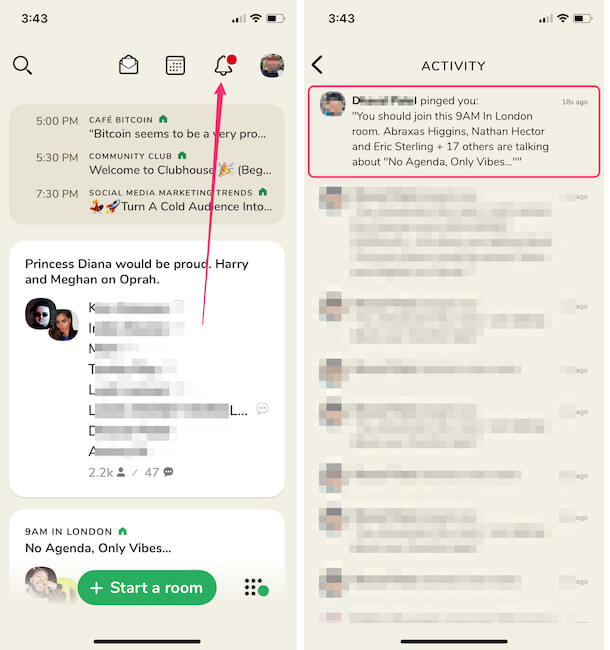**Detailed Image Caption:**

The composite image showcases two side-by-side screenshots of an application with a beige background, possibly a social or discussion platform similar to Discord.

The left screenshot appears to feature multiple sections and notifications of various events and updates. At the top, a calendar or agenda lists events for the day:
- 5:00 p.m.: Cafe Bitcoin
- 5:30 p.m.: Community Club
- 7:30 p.m.: Social Media Marketing Trends

Below the agenda, there's a headline reading, "Princess Diana Would Be Proud: Harry and Meghan on Oprah," followed by a block of blurred-out text. As you scroll further down, another time-based note reads, "9 a.m. in London, No Agenda." At the bottom of the left screenshot, there's a prominent green button labeled "Start a Room," suggesting the possibility of initiating a discussion or chat room. An unread notification icon is also visible, indicating new activity or messages.

The right screenshot seems to display recent activities and interactions. At the top, it shows, "Activity: Someone pinged you. You should join this 9 a.m. in London room." The room discussion involves individuals named Abraxas Higgins, Nathan Hector, and Eric Sterling, focusing on the topic "No Agenda Only Vibes." Below this notification, there are additional, but blurred, messages suggesting ongoing conversations or notifications.

Overall, these screenshots together indicate an application designed for scheduling events and facilitating community discussions, with features allowing users to create and join rooms for various topics and activities.